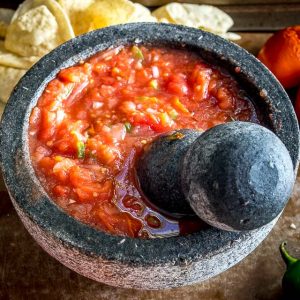The image showcases a close-up view of a stone gray mortar and pestle set, positioned on a brown wooden table. The mortar, which is round and matches the gray color of the pestle, contains a vibrant, chunky tomato salsa. The salsa features prominent red tomato pieces, shiny liquid, and noticeable bits of green jalapeños. The pestle, which is inserted into the salsa, appears to have been used for breaking down the ingredients, creating a texture that is part chunky and part smooth. In the upper left corner of the image, there are light-colored tortilla chips visible, ready to be dipped into the salsa. Additionally, in the upper right and lower right corners, green jalapeños make an appearance, with a green pepper stem distinctly visible in the lower right. The overall setup emphasizes the homemade, freshly-prepared nature of the salsa.